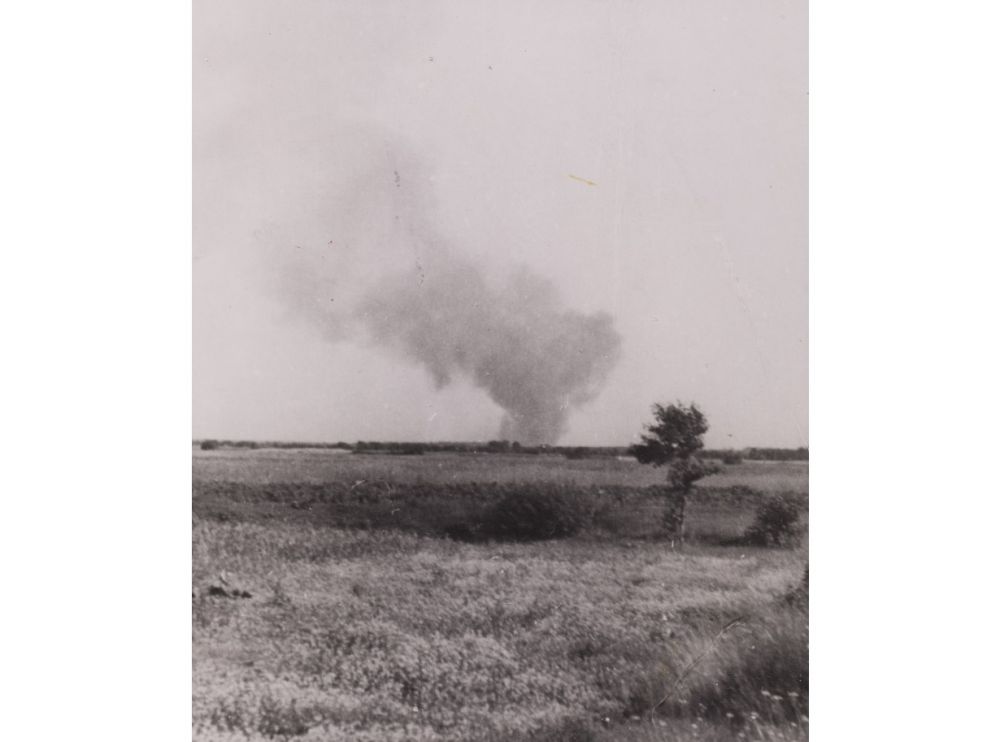This detailed black-and-white photograph captures a dramatic scene of a distant bushfire. A substantial plume of smoke rises ominously from the central horizon, billowing into an empty, white sky devoid of any visible clouds. The foreground of the image features a grassy plain, interspersed with scrubby bushland and patches of long, wispy plants that resemble wheat or weeds, possibly adorned with white flowers. Towards the lower right of the frame stands a solitary tree, its alignment seemingly influenced by the directional flow of the smoke. The terrain includes darker, shadowy areas that suggest slight elevation changes, adding texture to the continuous field. Near the horizon, a dim, darker strip could indicate the presence of distant trees or man-made structures, subtly emphasizing the fire's reach across the landscape.